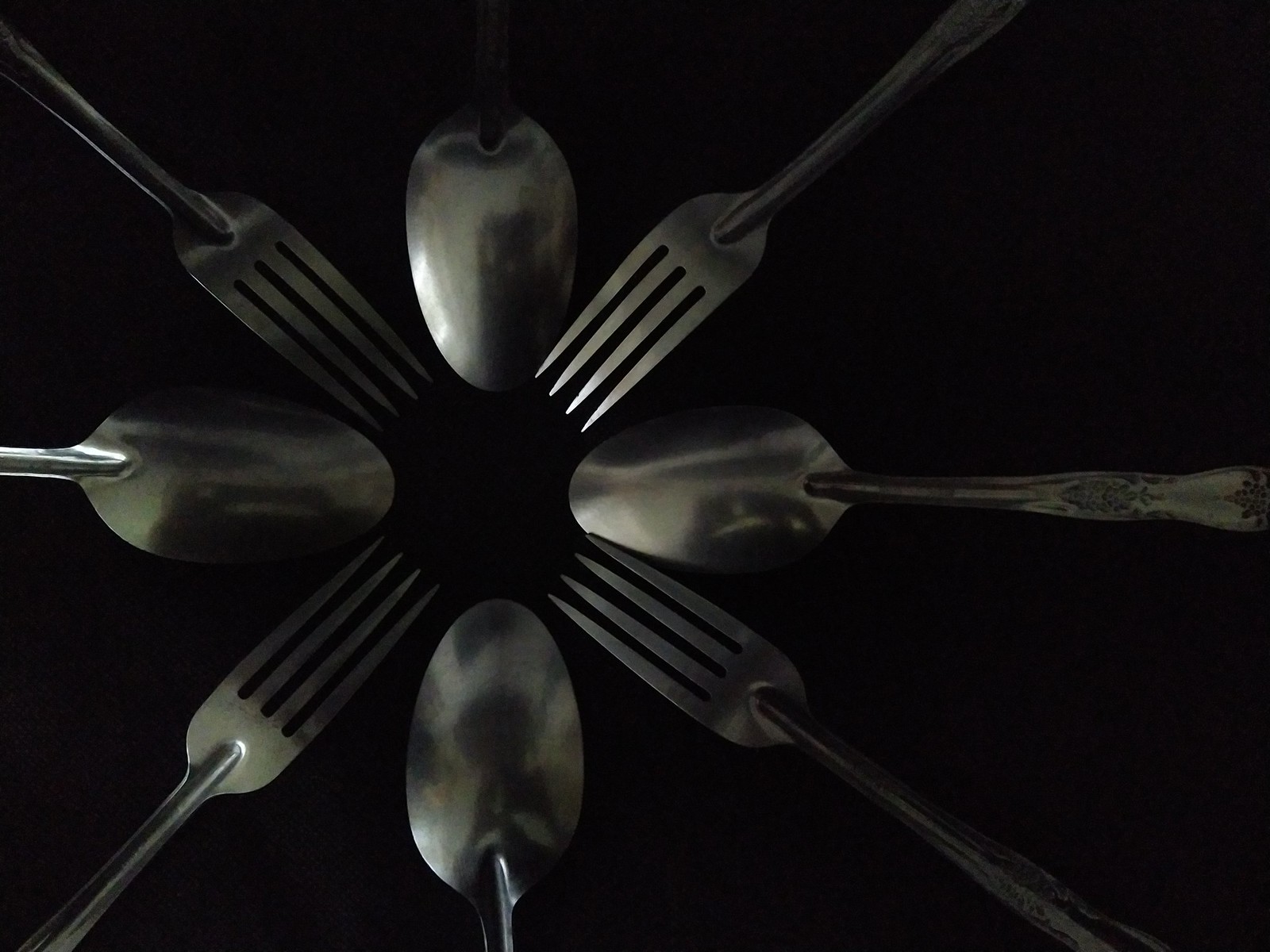This horizontally rectangular image set against a featureless black background showcases a meticulously arranged circle of alternating silver metal spoons and forks, forming a rosette or star pattern. There are four spoons and four forks, all pointing their handles outward from the center. The utensils are slightly off-center to the left, with the upper surfaces turned downward, showing their convex curves. The spoons have flower-like designs on their handles, which flair in and out before narrowing at the base of the round, glistening portion. The shimmering forks, with their straight handles, are interspersed between the spoons. The arrangement resembles a clock, with the 12 o'clock position occupied by a spoon and continuing in an alternating pattern. The silverware appears to be stainless steel, capturing light beautifully, and faint reflections, possibly of the photographer, can be discerned in a couple of the spoons.